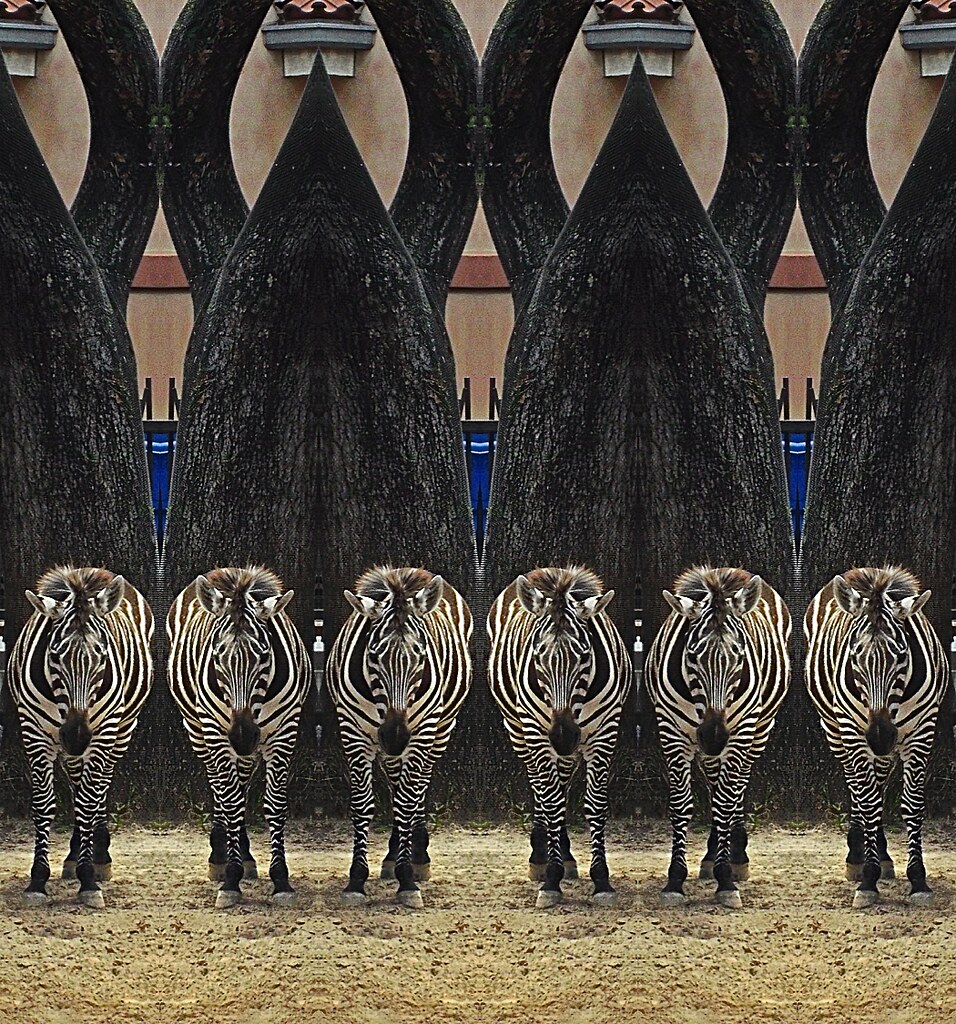This highly detailed image showcases six zebras, all identically marked with black and white stripes, standing evenly spaced in a straight row and facing directly towards the camera. The zebras, standing on a dirt surface sprinkled with small pebbles, exhibit darkened legs near their hooves, which are off-white. Behind them, the scene is framed by four tall, black, obelisk-shaped structures, resembling elongated teardrops or bullets that taper to a point at the top. These structures also have circular extensions at their peaks, somewhat like arms raised overhead. 

Interspersed between these stark, textured forms is a glimpse of bright blue, suggesting a backdrop that may be either the sky or a canopy. Further back stands a wrought iron fence, leading to a tan-colored building with a strip of dark brown molding and four semi-circular, sconce-like lights. The building itself has a somewhat terracotta tinge, adding a subtle warmth to the otherwise balanced and symmetrical composition. The illustration, possibly digital given its precise details and replicate nature of the zebras, combines elements of nature and architecture into a strikingly unusual yet coherent image.